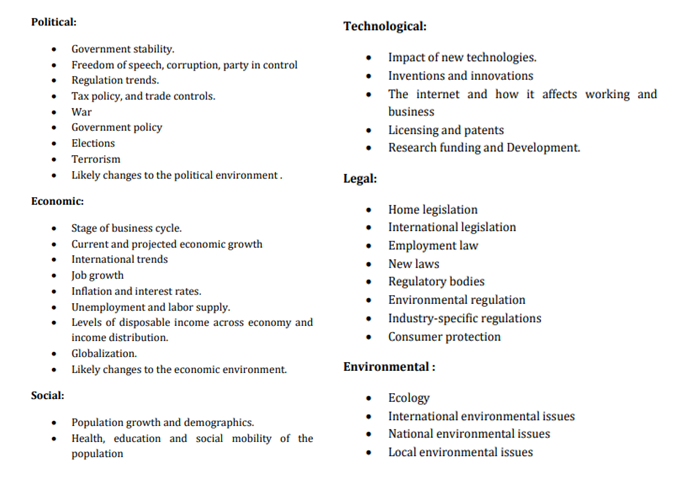This image displays a structured document organized into different sections based on various themes, such as Political, Economic, Social, Technological, Legal, and Environmental factors. Each section is introduced by a bold, larger font heading, followed by a list of related bullet points that detail specific topics.

- **Political:**
  - Government stability
  - Freedom of speech
  - Corruption
  - Political party regulations
  - Tax policies
  - War
  - Government policy
  - Elections
  - Terrorism
  - Likely changes

- **Economic:**
  - Stage of the business cycle (current and projected)
  - International trends
  - Job growth
  - Inflation
  - Unemployment
  - Labor conditions
  - Levels of disposable income
  - Several other factors

- **Social:**
  - Population growth
  - Health and education

- **Technological:**
  - New technology inventions and innovations
  - Impact of the internet on work and business
  - Licensing and patents
  - Research funding and development

- **Legal:**
  - Home legislation
  - International employment law
  - New laws
  - Regulatory bodies
  - Environmental regulations
  - Industry-specific regulations
  - Consumer protection

- **Environmental:**
  - Ecological issues
  - International environmental issues
  - Natural environment concerns
  - Local environmental issues

The document is visually organized in a monochromatic scheme, with headings set in a larger font for emphasis, and bullet points indented below each heading. This allows for clear delineation of topics within each category, facilitating ease of reading and comprehension.